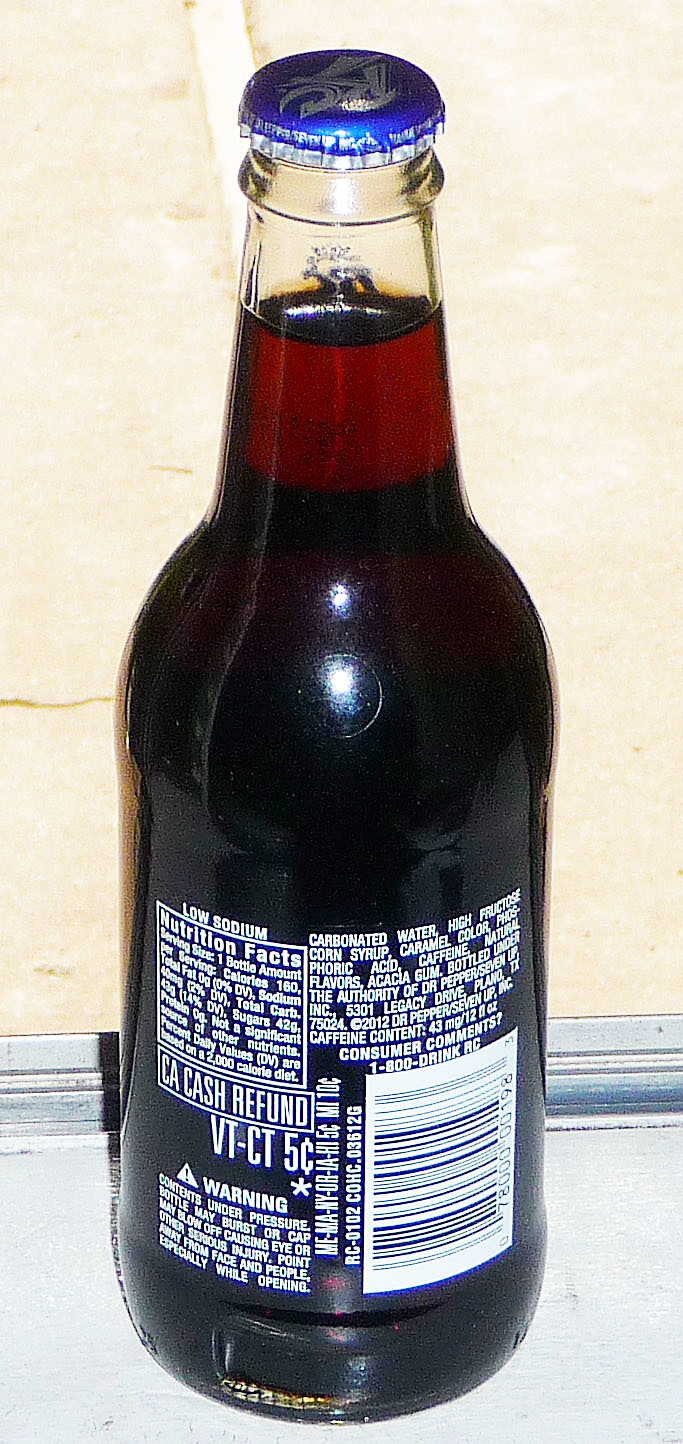A detailed caption for the described image could be:

"Displayed in the photograph is a classic glass bottle of RC Cola, positioned on a sleek gray surface. The backdrop includes a partial view of a metal divider and a tan tile floor accented with white grout, though the image is highly zoomed in, focusing primarily on the soda bottle. The beverage within the bottle is a rich brown color, characteristic of RC Cola. The bottle is capped with a distinctive blue pop cap featuring silver lettering that spells out 'RC'. The back of the bottle contains detailed information, including ingredients such as carbonated water, high fructose corn syrup, caramel color, phosphoric acid, caffeine, natural flavors, and acai gum. It is noted to be bottled under the authority of Dr Pepper/Seven Up, Inc., located at 5301 Legacy Drive, Plano, TX. Nutritional information indicates that the soda is low in sodium, with a serving size of one bottle amounting to 160 calories. Additional details mention a CA cash refund and a VTCT 5-cent deposit. A warning highlights that the contents are under pressure, cautioning that the bottle may burst or the cap may blow off, potentially causing eye or other serious injuries, advising to point away from the face or people when opening."